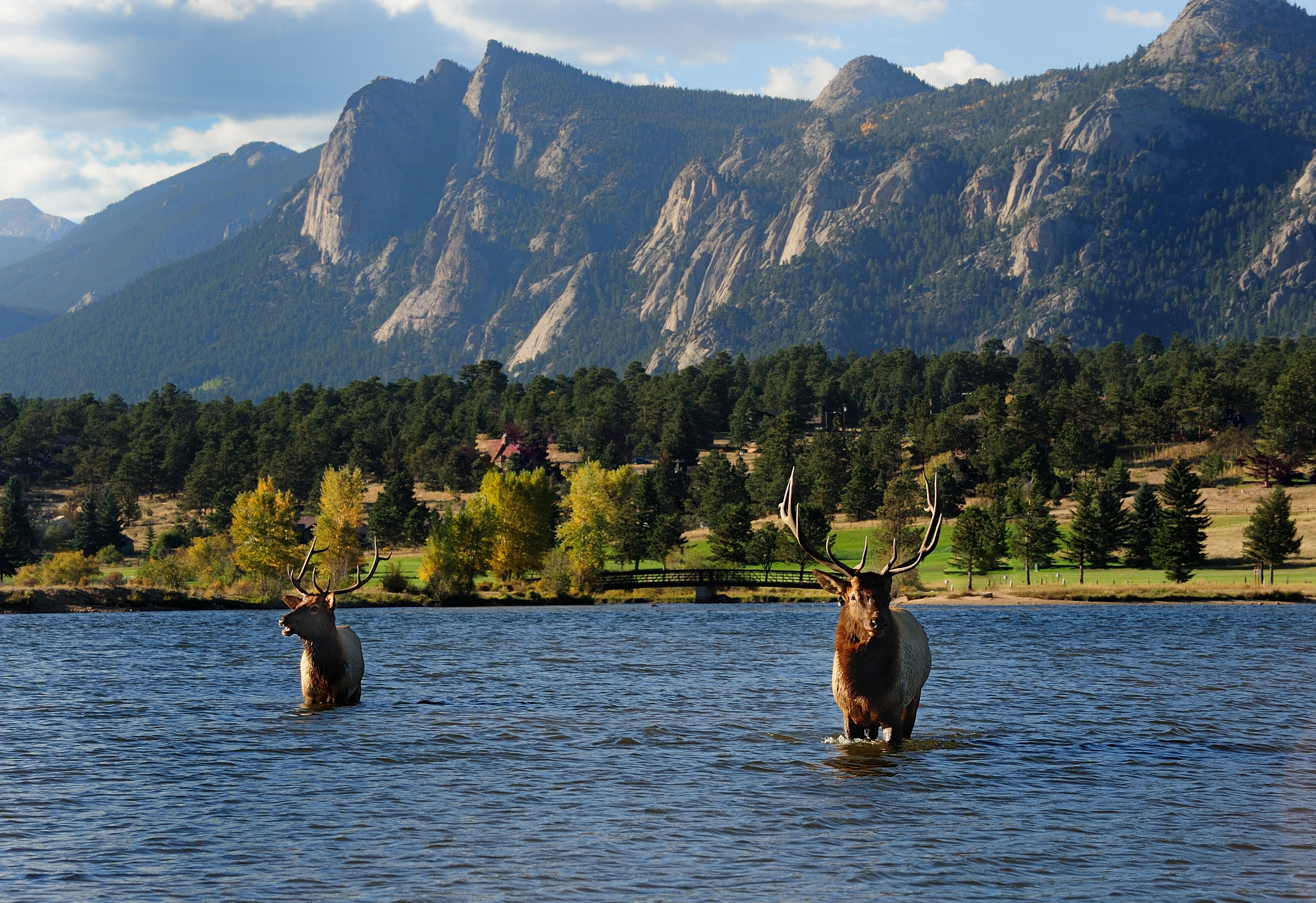In this high-resolution photograph of a bucolic wildlife landscape, two majestic elk, distinguished by their large antlers, stand in a serene, blue river. One elk, knee-deep in the water, faces the viewer with its mouth open slightly to the left, while the other, chest-deep, stares more directly at the camera. The elk on the right boasts furrier neck and larger antlers. The image is beautifully layered: the bottom third is dominated by the tranquil river water; the middle third showcases a tapestry of green land with a mix of dark green pine trees and lighter green vegetation, accompanied by a bridge; the top third is adorned with rugged, tree-speckled mountains beneath a clear sky. The landscape transitions smoothly from the vibrant watery foreground to the lush mid-ground, up to the majestic mountainous background, underscoring the pristine beauty of nature.